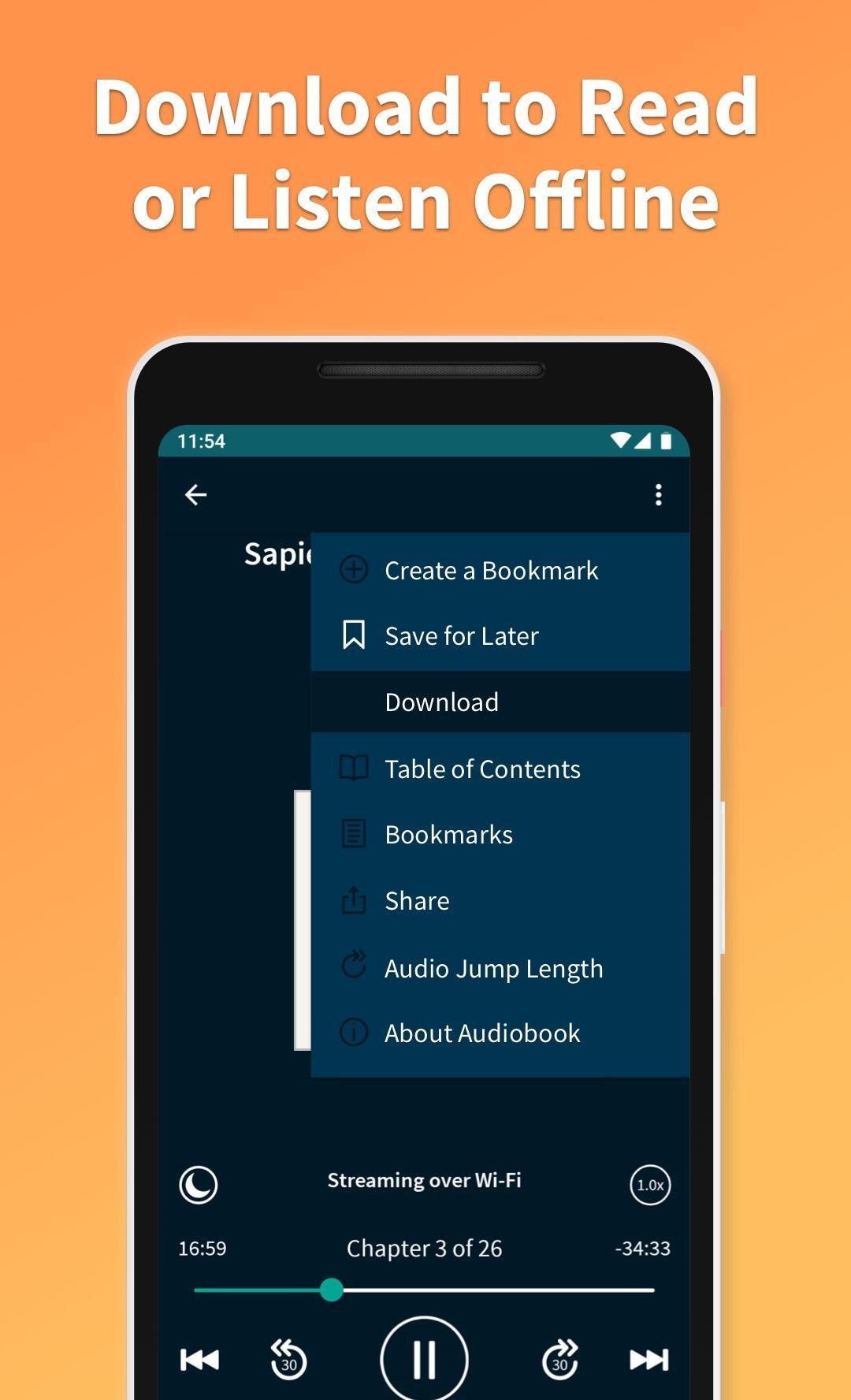**Caption:**
On an orange background, with the words "Download to read or listen offline" written in white letters, the image features a smartphone with a full battery and active WiFi connection. The time displayed is 11:54. Superimposed on the screen, a blue box is prominently featured in the foreground. This box includes options such as "Create a Bookmark" with a plus sign next to it, "Save for Later" with a save flag icon, and "Download," which is highlighted. Below these options, the box lists "Table of Contents," "Bookmarks," "Share," "Audio Jump Length," and "About Audiobook." At the bottom of the screen, a progress bar shows that the audio book is streaming over WiFi, currently at Chapter 3 out of 26. The playback time is 16 minutes and 59 seconds, with 34 minutes remaining in the chapter. In the background, additional elements are slightly obscured by the prominent foreground elements.